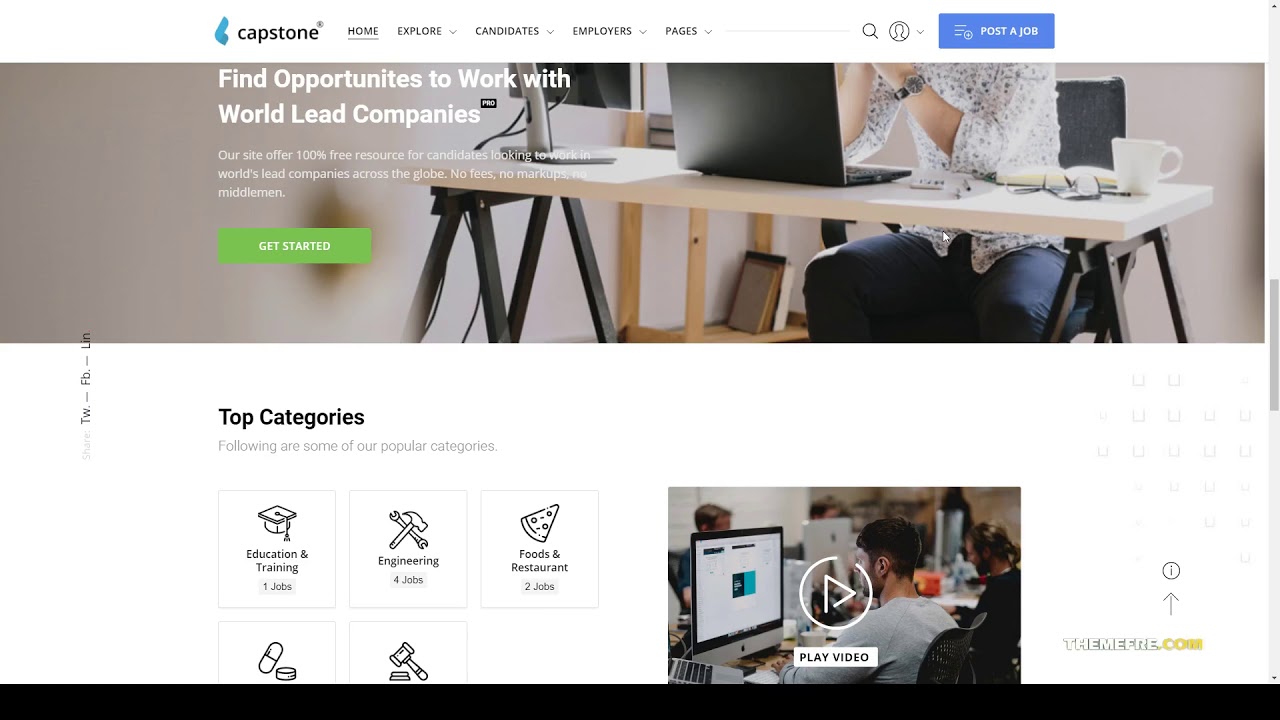The screenshot depicts a website's homepage. It is formatted horizontally with a sleek and organized layout. 

At the top left corner, there's a minimalist logo featuring the word "capstone" in black lowercase letters accompanied by a small, blue L-shaped icon. Adjacent to this logo, there's a horizontal menu bar with several options listed from left to right: Home, Explore, Candidates, Employers, and Pages. Notably, the "Home" option is underlined, indicating the current page. To the right of these menu options, there's a search bar followed by a prominent blue button labeled "Post a Job" in white text.

Spanning across the page below the menu is a large advertisement with a stock image background. The image showcases a person (whose head is not visible) sitting at a desk with an open laptop. Overlaying this image is a bold and inviting message in white text: "Good opportunities to work with world-leading companies." Below this, smaller text elaborates: "Our site offers 100% free resources for candidates looking to work in world-leading companies across the globe. No fees, no markups, no middlemen." At the bottom of this advertisement, there's a green rectangular button with the prompt "Get Started" in white text.

Further down the page, there is a section titled "Top Categories," introducing some of the popular job categories available on the site. The first three categories listed are Education and Training, Engineering, and Foods and Restaurants, though there are a total of five categories shown.

Overall, the screenshot reflects a user-friendly interface aimed at connecting job seekers with leading global companies, emphasizing accessibility and ease of use.